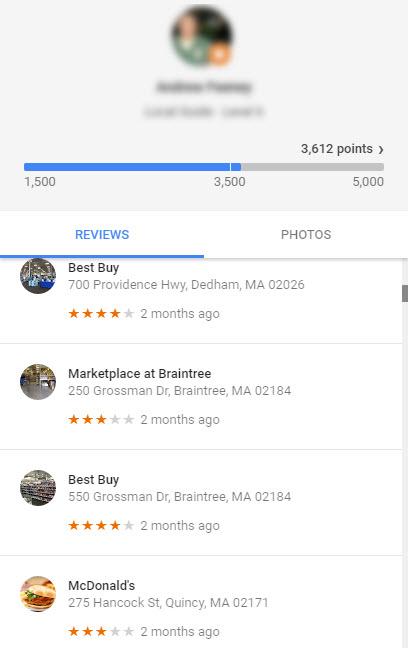Screenshot of a User's Profile Page with Reviews

This image is a screenshot of a slightly opaque profile page, featuring several blurred elements. At the center, a man is pictured wearing a green shirt layered over a white undershirt; however, his face and name are indistinguishable due to blurring. An orange circle containing a white circle can be seen within the image. 

Above the blurred man, there is a dark gray bar that displays the numbers 1500, 3500, and 5000. Towards the top right corner, in bold black text, it states "3612 points" accompanied by an arrow pointing to the right. A blue progress line extends slightly past the 3500 mark underneath these numbers. 

Below this section, the page has two tabs: "Reviews," which is underlined in blue, and "Photos" in gray. Under the "Reviews" tab, multiple review entries for various locations are listed, each featuring a small profile picture.

1. **Best Buy**  
   - Location: 700 Providence Highway, Dedham, MA 02026  
   - Rating: 4 out of 5 stars  
   - Review Date: 2 months ago  

2. **Marketplace at Raintree**  
   - Location: 250 Grossman Drive, Braintree, MA 02184  
   - Rating: 3 out of 5 stars  
   - Review Date: 2 months ago  

3. **Best Buy**  
   - Location: 550 Grossman Drive, Braintree, MA 02184  
   - Rating: 4 out of 5 stars  

4. **McDonald's**  
   - Location: 275 Hancock Street, Quincy, MA 02171  
   - Rating: 3 out of 5 stars  
   - Review Date: 2 months ago